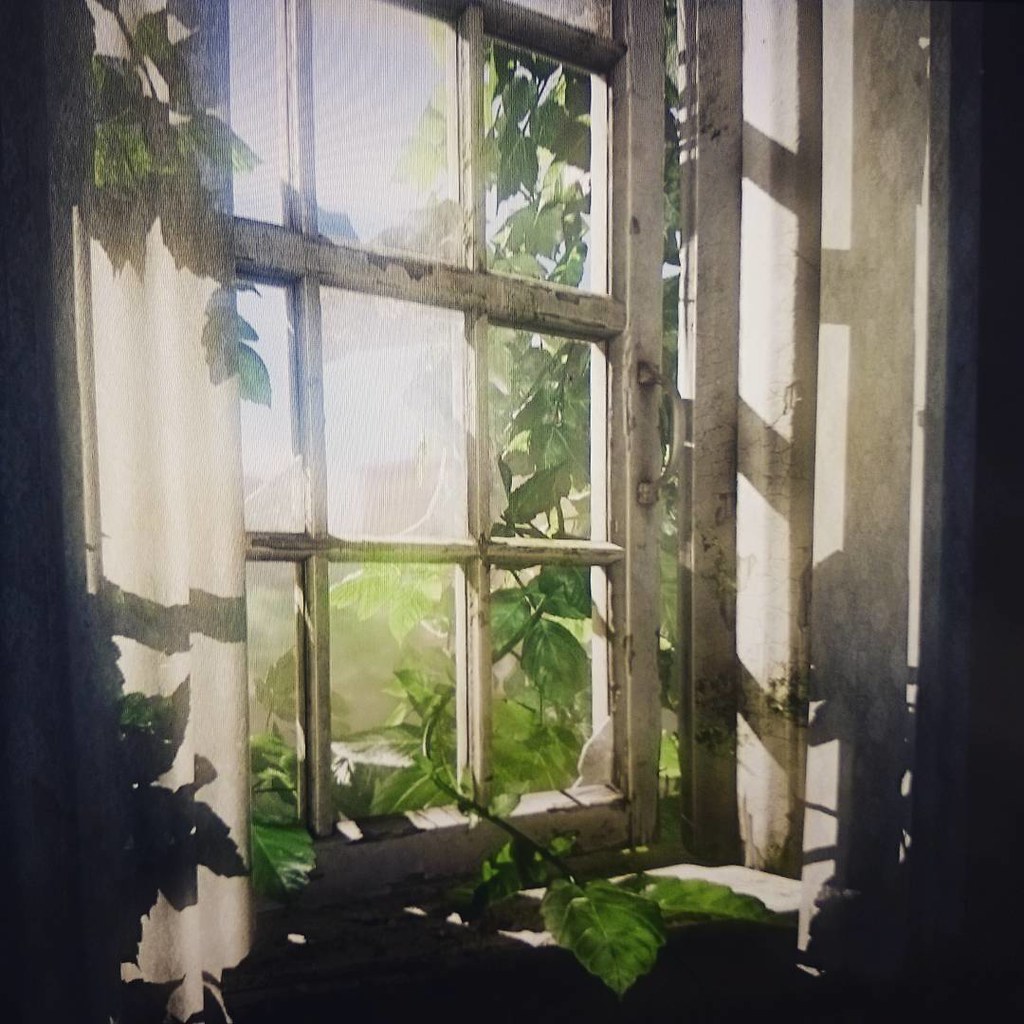A photograph that almost resembles a painting captures the serene view through an old-fashioned, multipane window composed of three panes across and four panes down. This charming window, which opens outward like a door and features a small handle, is partially adorned with curtains hanging on the left side. Outside, the sunlight illuminates the scene, casting shadows of leaves and the wooden grid of the window onto the right-hand wall inside. Enhancing the natural beauty, a vine with green leaves has made its way through the window, draping itself elegantly across the windowsill and mingling with its outer counterpart. The overall composition exudes a tranquil and timeless ambiance.